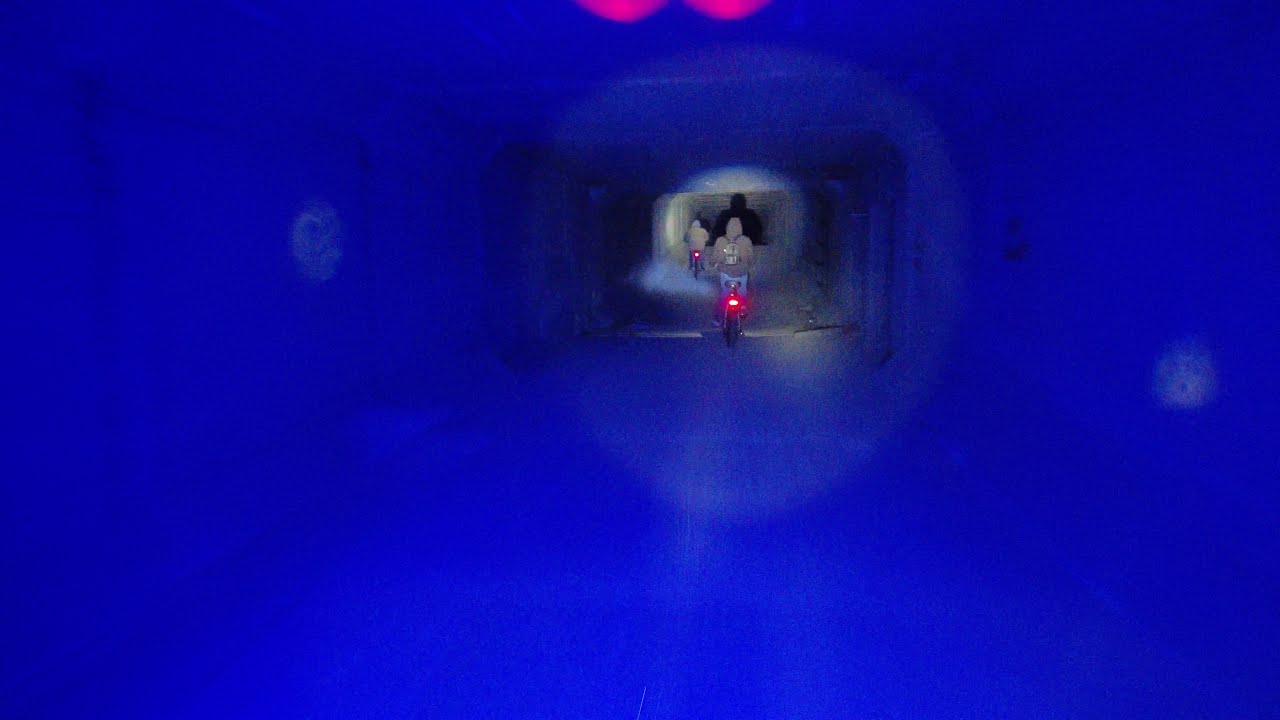The image captures a rectangular tunnel illuminated with a bright ultramarine navy blue light that envelops the entire space, casting a stunning glow on its walls. Within this futuristic corridor, two people are riding bicycles away from the viewer, deep into the tunnel's depths. The person closest to the center of the image is prominent, slightly to the right, wearing a gray hoodie and blue jeans, with a backpack featuring black straps that might be greenish in color. Just off to the left, above this person's left shoulder, is the second cyclist, slightly more distant yet still discernible. Both bicycles are equipped with glowing red taillights, which leave a haunting reflection on the dark, shadowy path ahead of them. The ambient blue light accentuates their attire—both are clad in hooded jackets that blend khaki gray hues with the ethereal luminescence of the tunnel. The cyclists are bathed in shadowy silhouettes as they ride towards the tunnel's vanishing point, creating a stark contrast against the vivid blue backdrop.